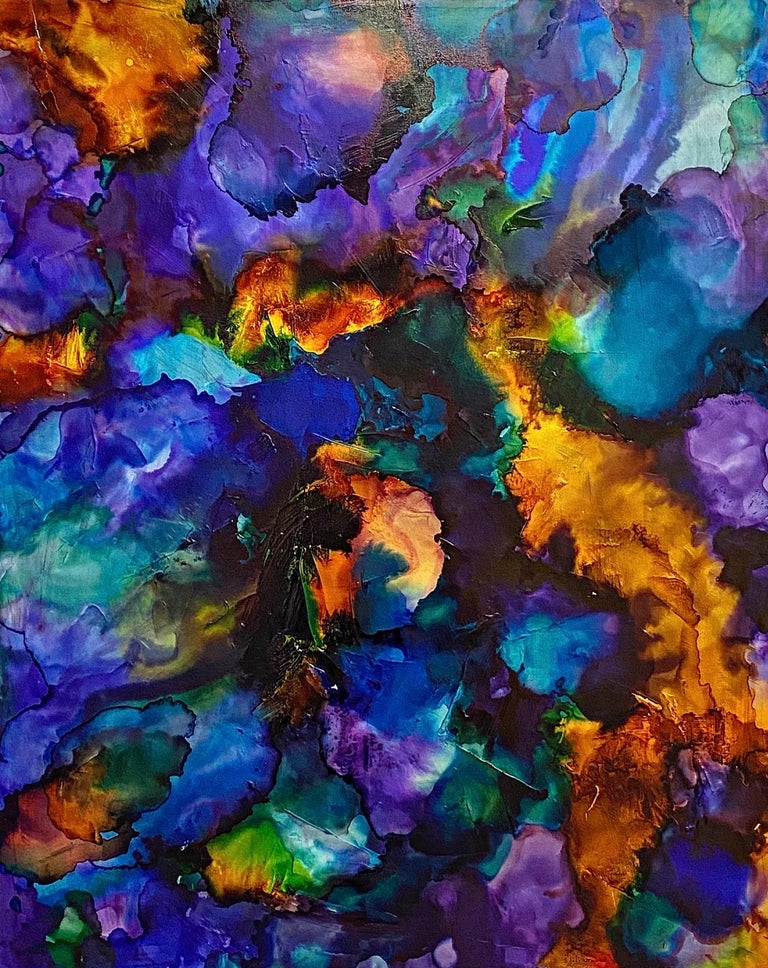This is a photograph of an abstract oil painting characterized by its chaotic and vibrant color scheme. The painting features a dynamic mixture of bright oranges, teals, blues, and purples, with flashes of yellow, red, and green creating a vivid and glowing effect. The splotches and irregular shapes of color lend a fractal-like quality to the composition, though no recognizable objects or scenes are depicted. Heavy paint strokes add texture, enhancing the contrasts between dark spots and brilliantly colored areas. The complex interplay of hues and the lack of definitive forms make the painting a captivating and pleasant visual experience.